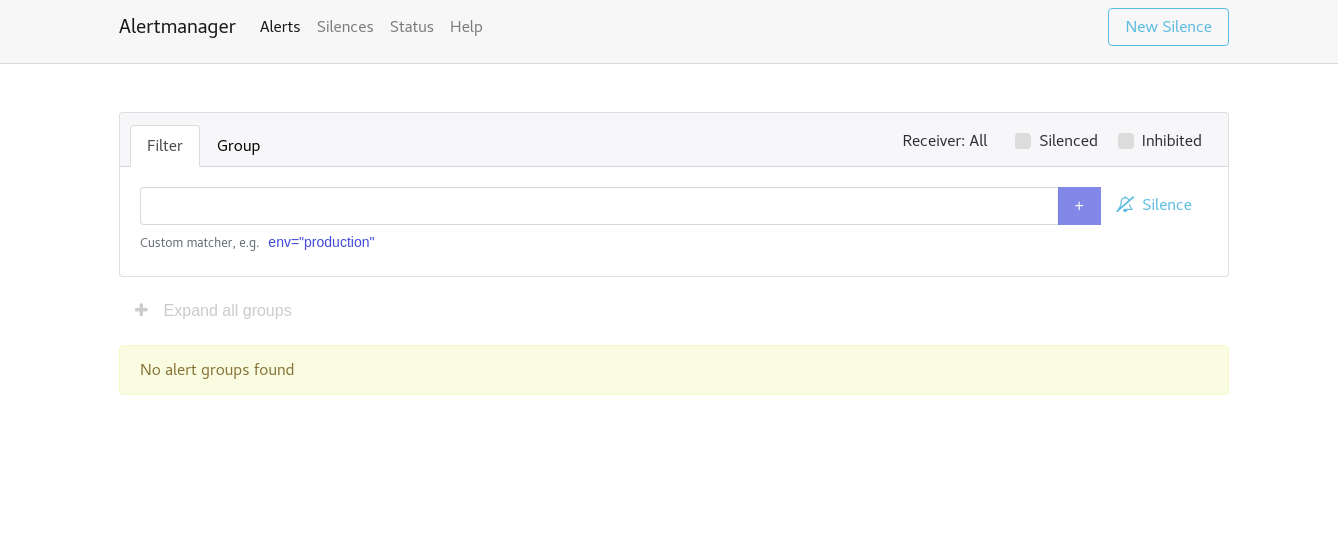The image is a horizontally rectangular screenshot of a web application's interface. At the very top, there is a light gray horizontal border. On the left-hand side of this border, in bold text, it reads "Alert Manager." Adjacent to this, there are several option tabs labeled "Alerts," "Silences," "Status," and "Help." On the right-hand side of the top border, there is a light blue square button with the text "New Silence" in light blue.

Below this top section, there is another horizontally rectangular section with a light gray banner at the top. This banner contains two tabs on the left side: "Filter" and "Group." The "Filter" tab is currently selected. On the right side of this banner, there is a dropdown that says "Receiver All," along with checkboxes for "Silenced" and "Inhibited."

Beneath the "Filter" tab, there is a text field where users can type in criteria, accompanied by a plus sign button. Below this text field, in small print, it reads "Custom Matcher: ENV = 'Production'."

Further down, there is an option labeled "+ Expand All Groups." Finally, at the very bottom, there is a pale yellow horizontal banner. On the left side of this banner, it states "No Alert Groups Found."